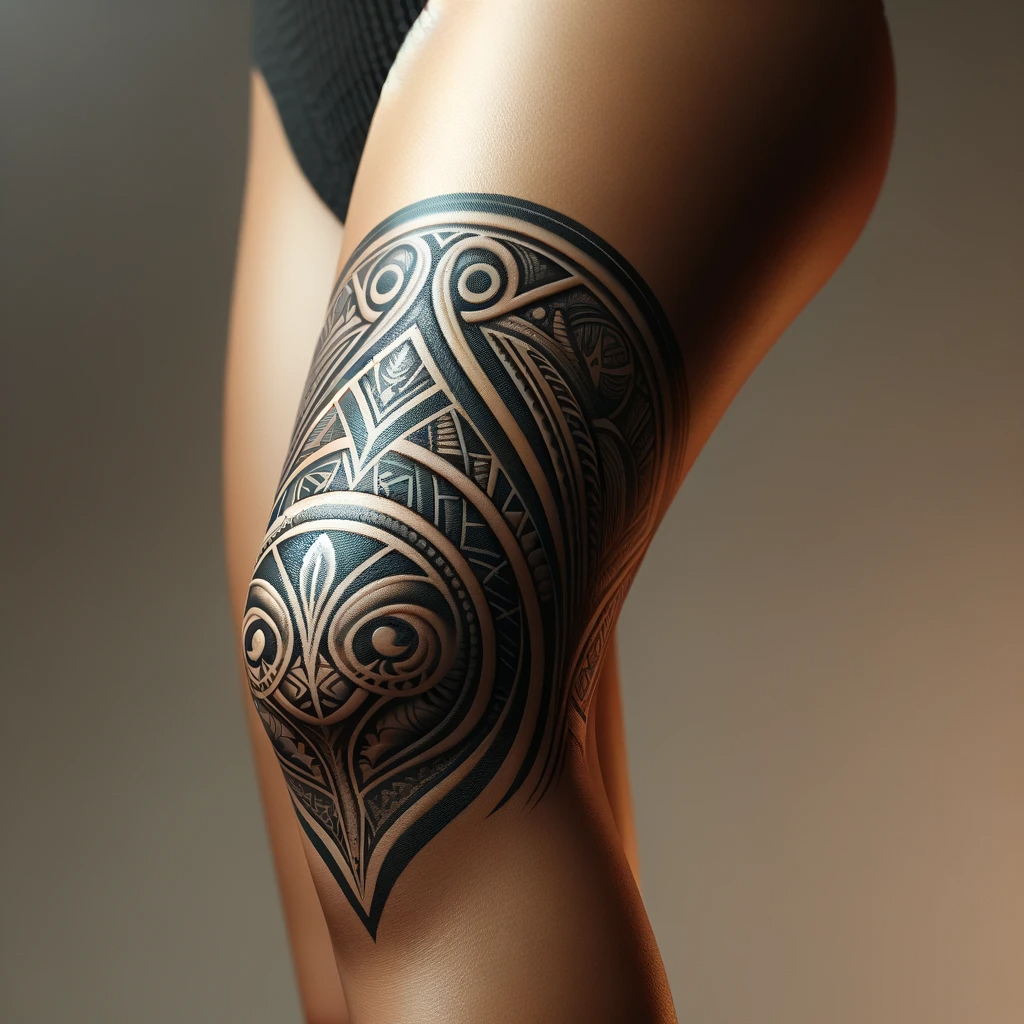The image features an AI-rendered depiction of a woman's legs, showcasing an intricately detailed, traditional black and grey tribal tattoo. Set against a dark, slightly fuzzy background, the woman's lower body is positioned sideways with her left knee slightly bent towards the camera. She is wearing black underwear, and the tattoo art extends from just below her knee up to her mid-thigh, wrapping around her leg. The tattoo incorporates elements reminiscent of Polynesian and Maori styles, including swirling patterns and ornate line work. At the knee, the design features a central circular motif with two prominent swirls, giving an impression of an owl's face or a fly's head, with lines and leaf-like details extending downwards and upwards around the leg. The smooth, shiny appearance of her legs and the high-quality rendering make the art stand out vividly against the background.